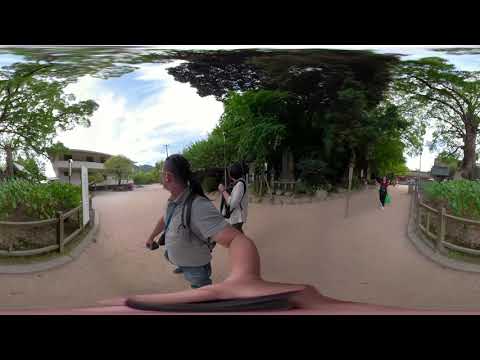The image depicts a vertical rectangular scene with a man on a tan sidewalk bordered by abundant greenery, including trees and shrubbery fenced off by short wooden rails. The man, positioned just left of center and facing away from the camera, has dark short hair and wears a gray short-sleeve shirt with blue jeans. He extends his hand toward the camera, which has been artistically blurred to stretch across the bottom of the picture. Additionally, the top of the image is blurred and curves inward, giving a distorted effect. In the background, a woman wearing a white shirt, dark pants (or a dark dress), and carrying a dark purse is also turned away. Both individuals seem to be walking near an intersection of various lanes in a town-like setting, which is bathed in bright, pleasant light. Low resolution adds a soft, almost nostalgic quality to the image, with numerous trees and some buildings in the distance. A green bag is faintly visible, adding a pop of color amid the predominantly green and neutral tones.